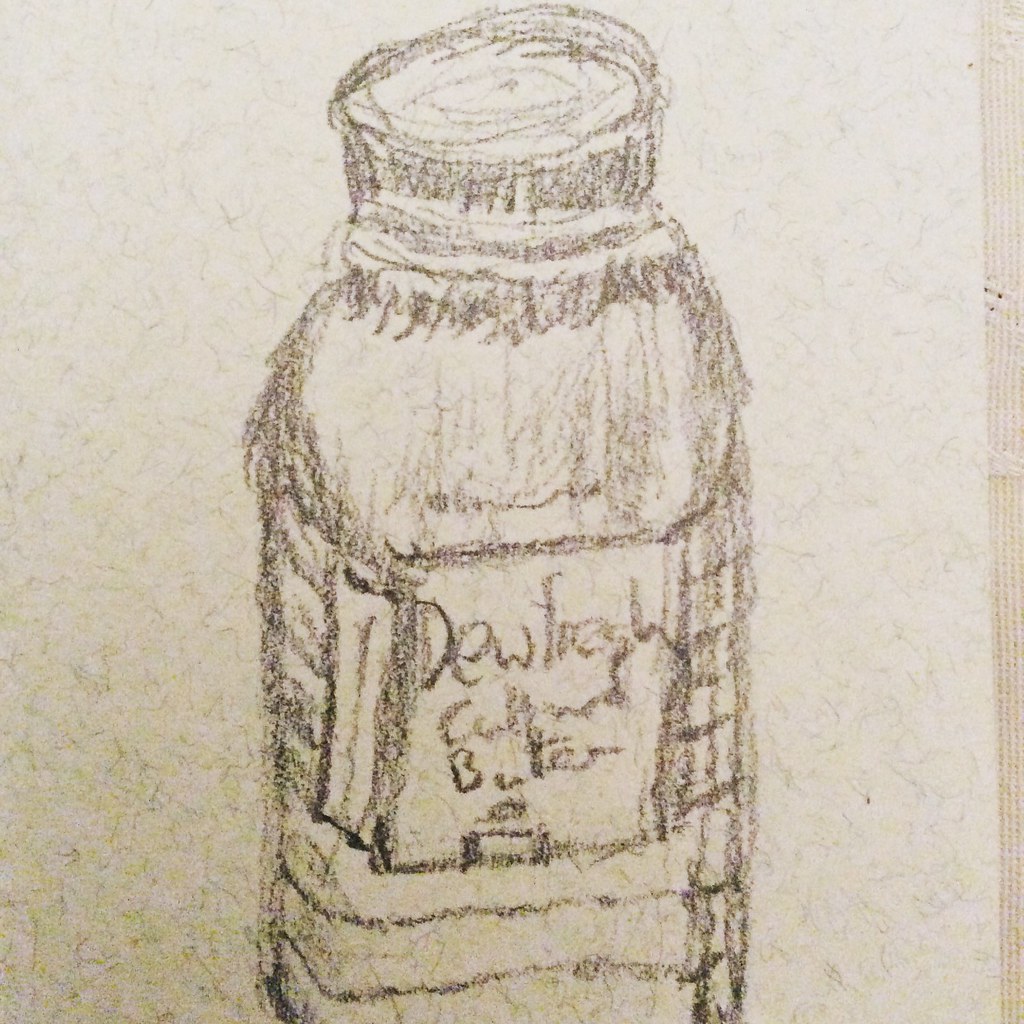This detailed pencil drawing on white paper features a bottle with a hand-drawn label. The label, although somewhat difficult to read, appears to say "Dew Fresh Cultured Butter." The bottle's cap resembles that of a milk bottle, with irregular, ragged lines suggesting it might be made of paper. Surrounding and beneath the label are distinct horizontal lines. The background of the drawing paper has a mottled texture, adding depth and a sense of authenticity to the artwork.